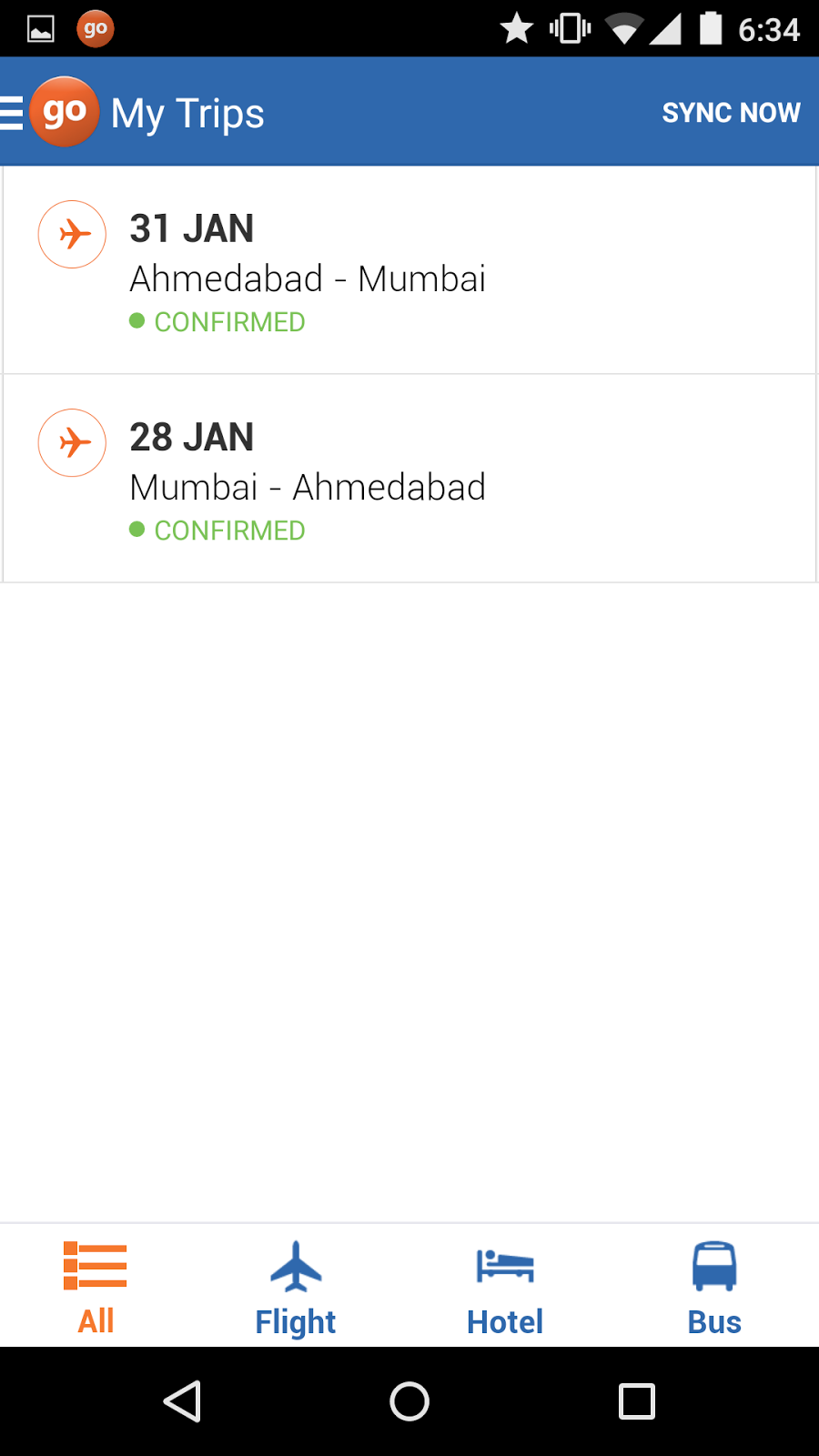The image depicts a screenshot from a user's cell phone. At the top of the screen, there is a graph, an orange circle with the word "GO" in white print, and several status icons including a star, a connectivity icon depicted as a triangle, a fully charged battery icon, and the time which reads 6:34. 

Underneath this section, there is a long, thin, blue rectangle with three white horizontal bars on the left side, next to another orange circle with the word "GO" in white. Inside this blue rectangle, in white print, is the text "MY TRIPS." On the far right of this rectangle, there is a "SYNC NOW" button, with the text displayed in all capital letters ("SYNC NOW").

Further down, there is a circular airplane icon followed by text indicating "31 January, Mumbai" along with a notification in green with a white circle stating "CONFIRMED." Another note mentions "Confirmed" again on January 28th. At the very bottom, there are additional emblems and a black rectangle.